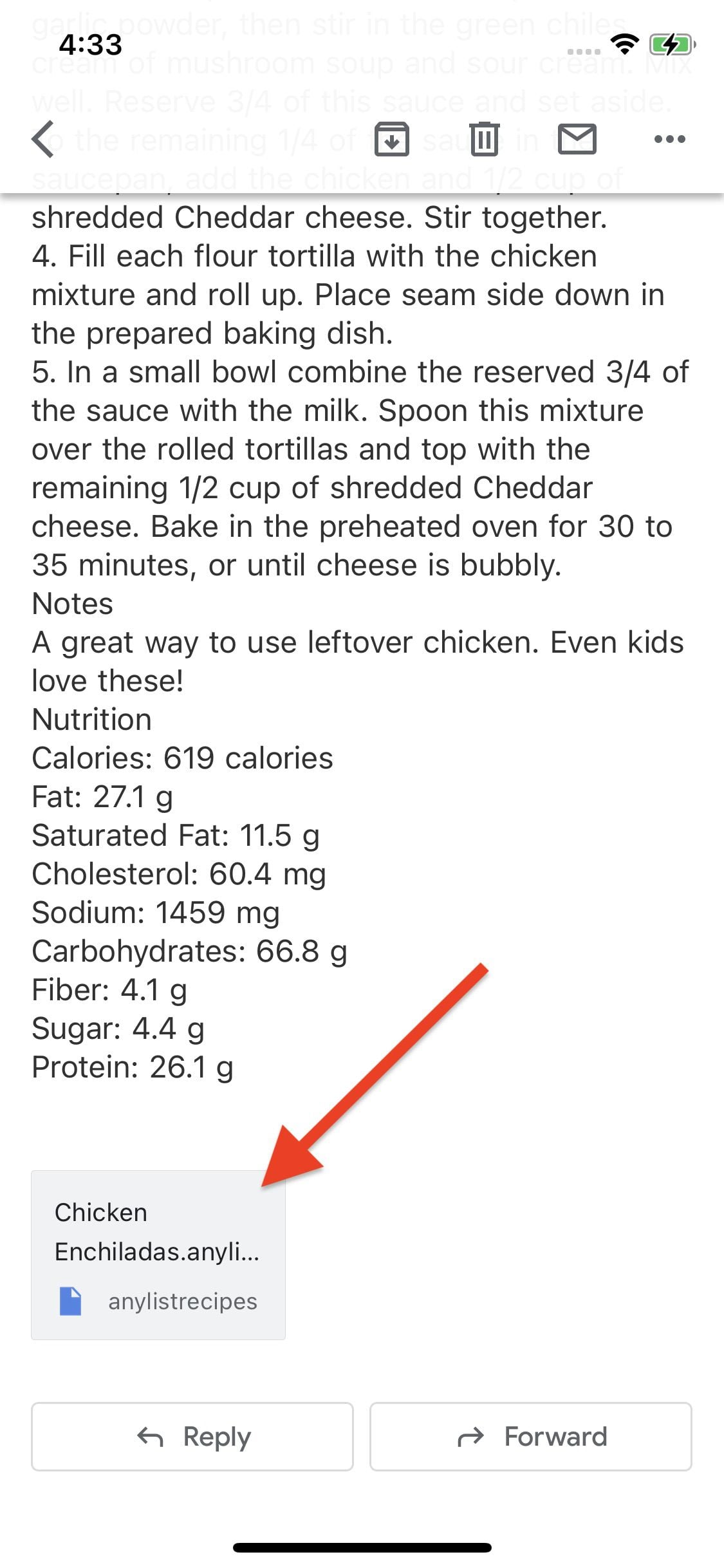In this image, there is a screenshot of an email displayed on a smartphone. The top part of the screen shows the time as 4:33 and a battery icon on the top right, which is green and indicates it's charging. Next to the battery icon is a Wi-Fi icon.

The email itself includes several actions like archive, delete, and inbox. The top portion of the email is slightly blurred, but the text is written in black. The email content appears to be a recipe and reads as follows:

"Garlic powder. Then stir in the green chili, cream of mushroom soup, sour cream, and shredded cheddar cheese. Stir together. Fill each flour tortilla with the chicken mixture and roll up. Place seam side down in the prepared baking dish. Then, in a small bowl, combine three-quarters of the remaining sauce with the milk. Spoon this mixture over the rolled tortillas and top with the remaining half cup of shredded cheddar cheese. Bake in the preheated oven for 30 to 35 minutes or until the cheese is bubbly. Note: This is a great way to use leftover chicken. Even kids love these. Nutrition: 619 calories, fat 27.1 grams, saturated fat 11.5 grams, cholesterol 60.4 milligrams, sodium 1459 milligrams, carbohydrate 66.8 grams, fiber 4.1 grams, sugar 4.4 grams, protein 26.1 grams."

There is a file attached to the email, located at the bottom left side of the screen, labeled "Chicken and Chili Enchiladas" along with a list of other recipes. A red arrow points toward this file. Additionally, there are visible reply and forward buttons.